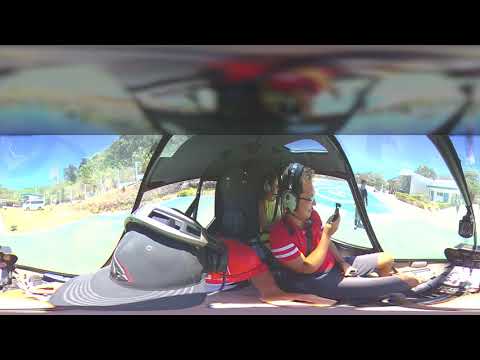In this vividly detailed outdoor scene, a man sits prominently in the center of a vehicle, captured as he looks to the right while engrossed in his phone. Dressed in a red t-shirt with white-striped short sleeves and light gray shorts, he wears a pair of headphones. The vehicle, possibly a helicopter, has a solid black border framing the scene, with a gray baseball cap resting on the dashboard in the front foreground. Just behind the man on his right, a woman in a yellow top gazes out of the window. Beyond the vehicle, there's a warm, outdoor setting featuring several buildings, green trees, and a strikingly clear blue sky. Scattered on the left are a few vehicles, while a colorful landscape, including distinct hues of black, green, red, purple, yellow, orange, tan, and gray, adds depth to the backdrop, resembling a picturesque day out.